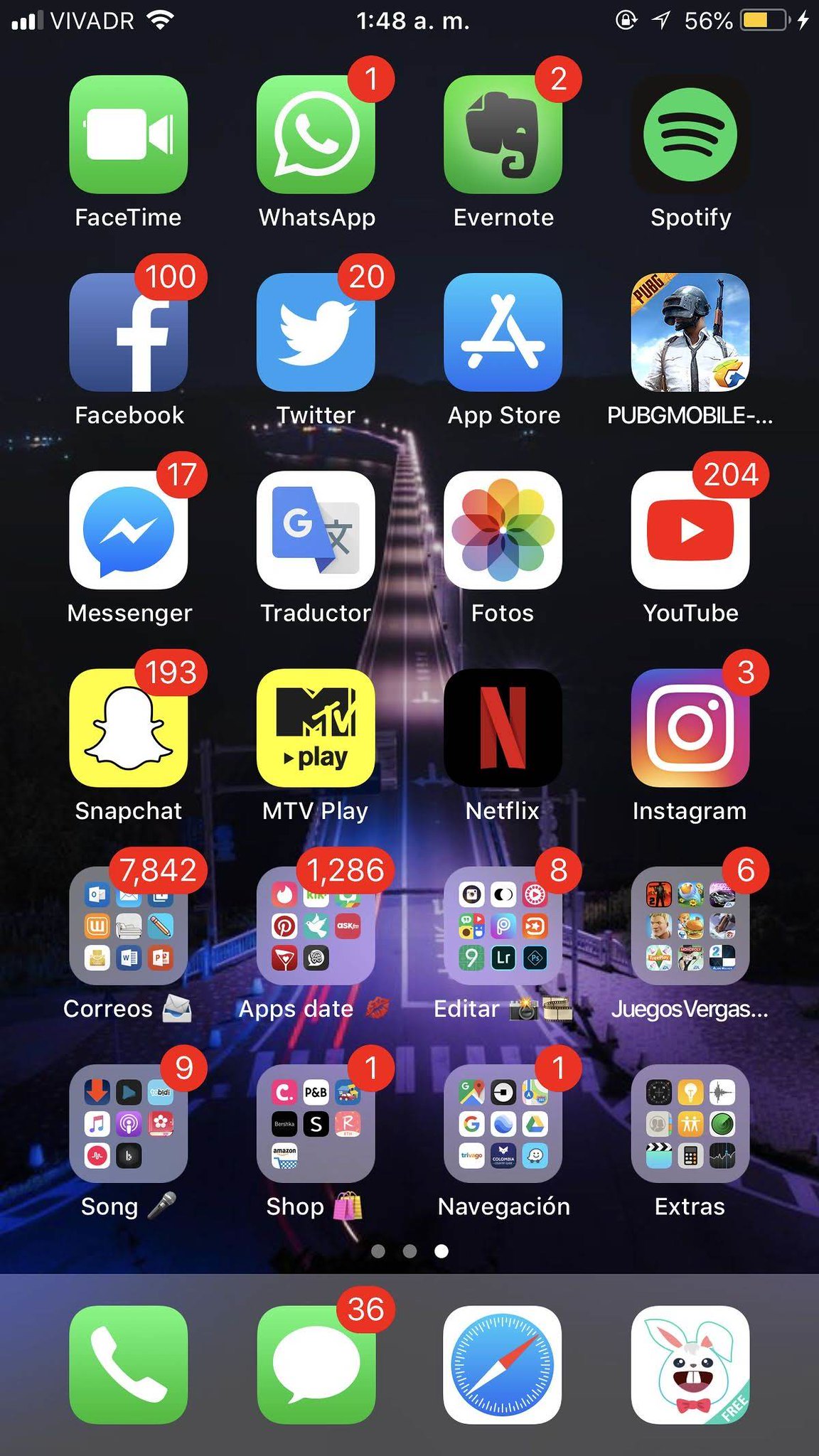A screenshot of a smartphone home screen is displayed, using a background that depicts a moody nighttime scene from a video game. The background features a long, curving road or bridge illuminated by streetlights, with shades of gray, blue, and black dominating the image. The contrast between the brightly lit streetlights and the surrounding dark environment emphasizes the nighttime setting.

The home screen is populated with 24 app icons organized into six rows. The apps include, from top left to bottom right: FaceTime, WhatsApp, Evernote, Spotify, Facebook, Twitter, App Store, PUBG Mobile (featuring an image of a person with a gun and a mask), Messenger, Traductor, Photos, YouTube, Snapchat, MTV Play, Netflix, Instagram, and several folders containing collections of apps labeled as Correos, App State, Editar, Juegos Vergas, Song, Shop, Navigacion, and Extras.

At the bottom of the screen, four frequently used apps are docked: the Phone app, the Messaging app (with a green background), Safari, and an app featuring a white background with a cartoon bunny wearing a bowtie.